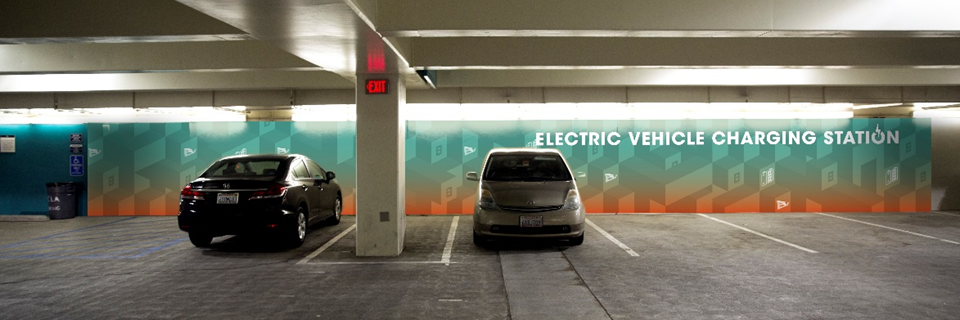In this image of a parking garage, there are two parked vehicles - a dark-colored sedan facing the wall and a light brown or tan van facing the viewer. The sedan occupies a handicap spot identified by a blue marking on the ground, while the van is in a regular parking spot. The van is positioned near the left side of the image, with several empty parking spaces to its right. Above these empty spaces, white text on the wall reads, "Electric Vehicle Charging Station," though no charging equipment is visible. The wall behind the cars features a vibrant mural with a blue-to-orange gradient depicting rectangular, building-like objects. To the left of the mural, a red exit sign is mounted on a pillar, which may also have an outlet. Nearby, a garbage can is placed against a slightly greenish-blue section of the wall. Far in the distance, there are indistinguishable black and blue signs. The garage appears empty, with no people present.